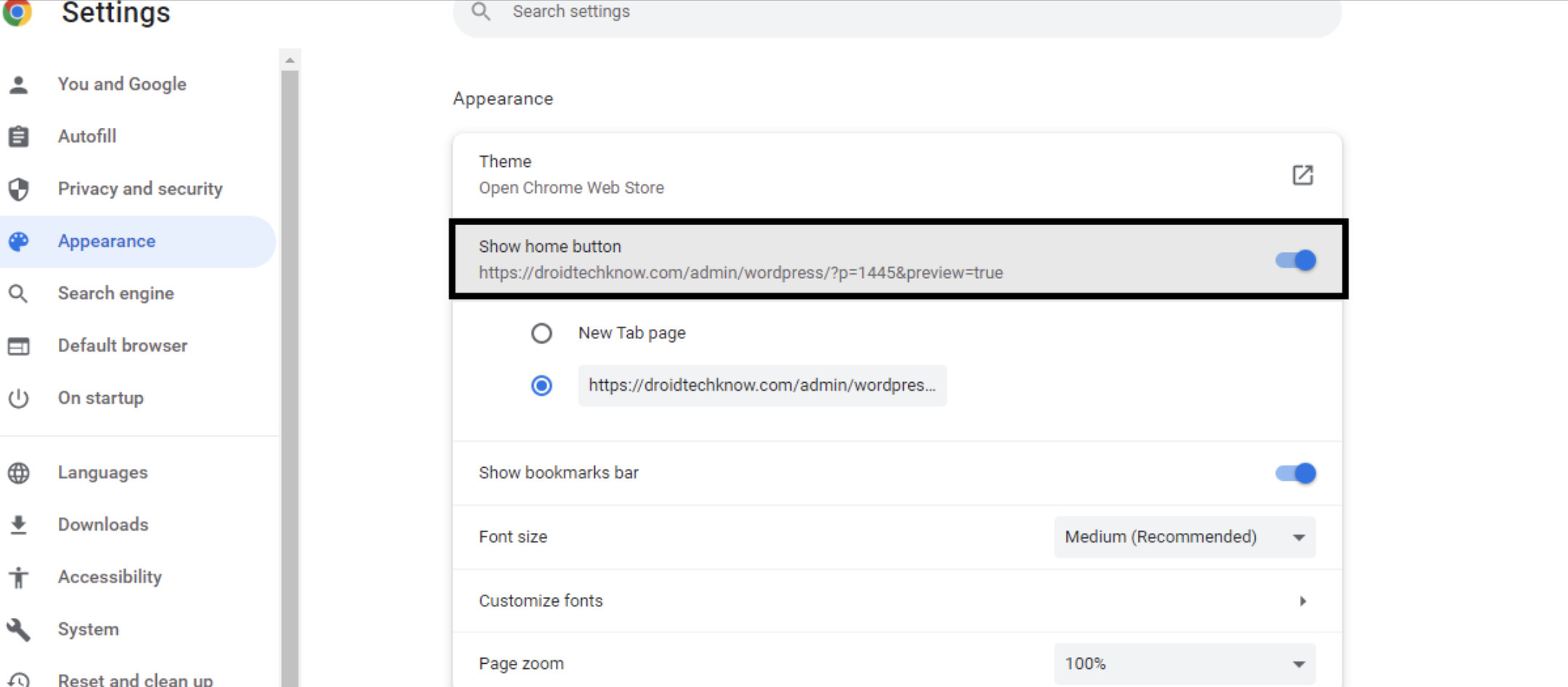This screenshot captures the "Settings" page of Google Chrome, with a black font label "Settings" located in the upper left corner, adjacent to the Google Chrome logo. Beneath the "Settings" label, there is a vertical navigation menu comprising several options: "You and Google," "Autofill," "Privacy and security," and "Appearance." The "Appearance" section is selected, highlighted in blue font with a light blue background.

In the main window, the "Appearance" settings are displayed. The first option in this section is "Theme," which includes a link to "Open Chrome Web Store to install any theme." 

Following this, there's a black outline indicating that the "Show home button" feature is turned on, with a toggle switch enabled. The specified web address for the home button is "droidtechno.com/admin/WordPress." Below that, the "New tab" page option is also toggled on, displaying the same web address.